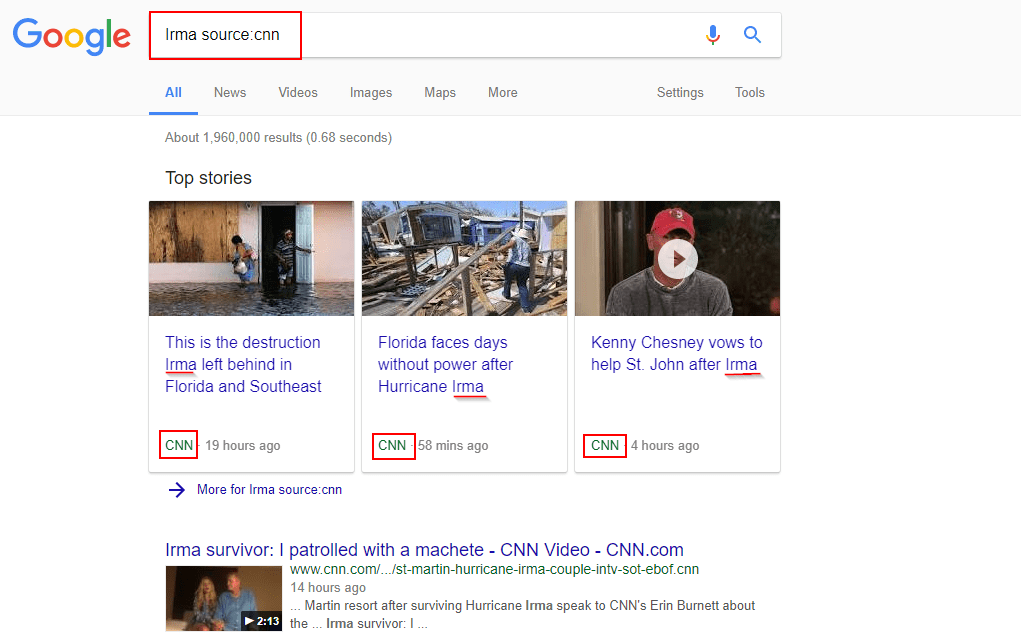This image depicts the Google search results page. Dominating the top left is the iconic Google logo, featuring the traditional color scheme of blue, red, yellow, blue, green, and red letters. To its immediate right is the search bar containing the text "Irma Source: CNN," encased in a red rectangular border. Adjacent to the search bar, on the far right, are two icons: a microphone and a magnifying glass, representing voice search and the search function, respectively.

Beneath the search bar is a navigation menu, beginning with the "All" category highlighted in blue text and underlined. Other visible categories include "News," "Videos," "Images," "Maps," and "More," followed by "Settings" and "Tools" on the far right. Further down, the page shows that there are approximately 1,960,000 results found in 0.68 seconds.

Centered under this information is the heading "Top stories," accompanied by three images. The first image is captioned "This is the destruction Irma left behind in Florida." The second image reads "Florida faces days without power after Hurricane Irma." The third image states "Kenny Chesney vows to help St. John after Irma." These images visually summarize the significant impact and ongoing repercussions of Hurricane Irma.